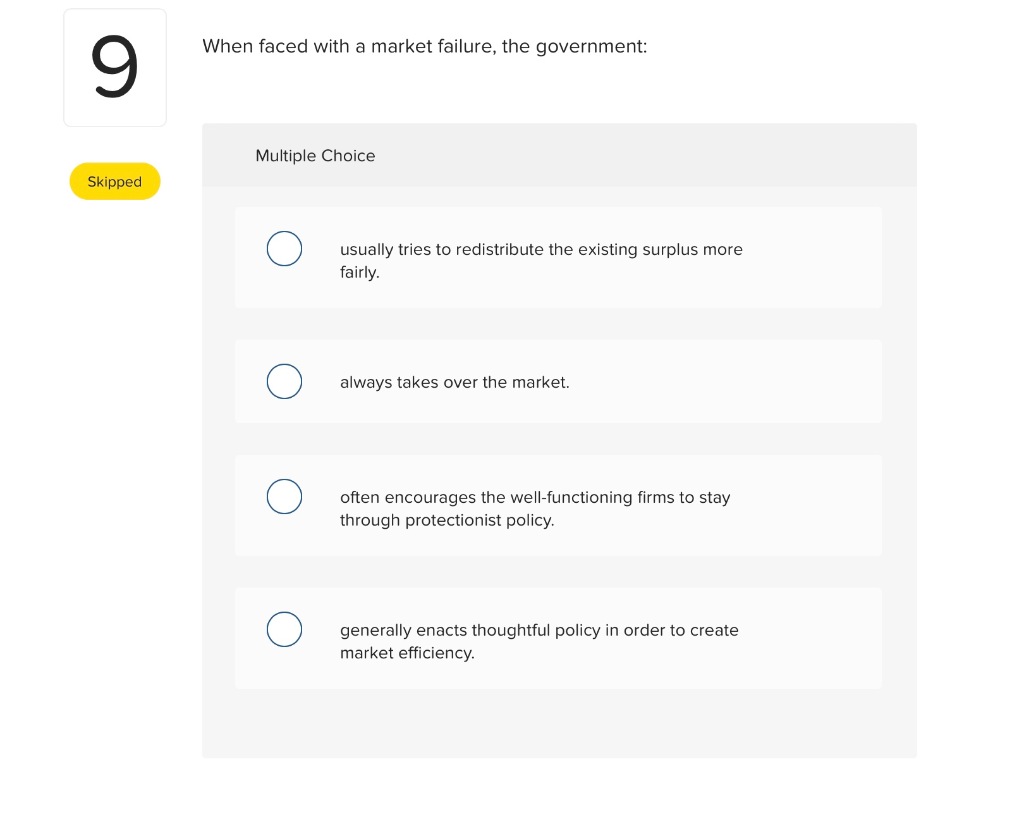This image showcases a website interface designed for a multiple-choice question. In the top left corner, there is a gray-outlined square with a white background, featuring a bold black number "9." Directly below this square, an oval-shaped yellow button with the word "Skipped" in black text stands out.

In the middle section of the page, a heading in black text reads: "When faced with a market failure, the government:" followed by a colon. Below this heading, also in black text, is the label "Multiple Choice."

The multiple-choice options are listed as follows:
1. An open circle next to the statement, "Usually tries to redistribute the existing surplus more fairly."
2. An open circle adjacent to the statement, "Always takes over the market."
3. An open circle alongside the statement, "Often encourages the well-functioning firms to stay through protection policy."
4. An open circle next to the statement, "Generally enacts thoughtful policy in order to create market efficiency."

Each option is clearly marked with a pre-set open circle for selection, and all text descriptions are in black. The layout is clean and structured, guiding the user to read and interact with the content seamlessly.